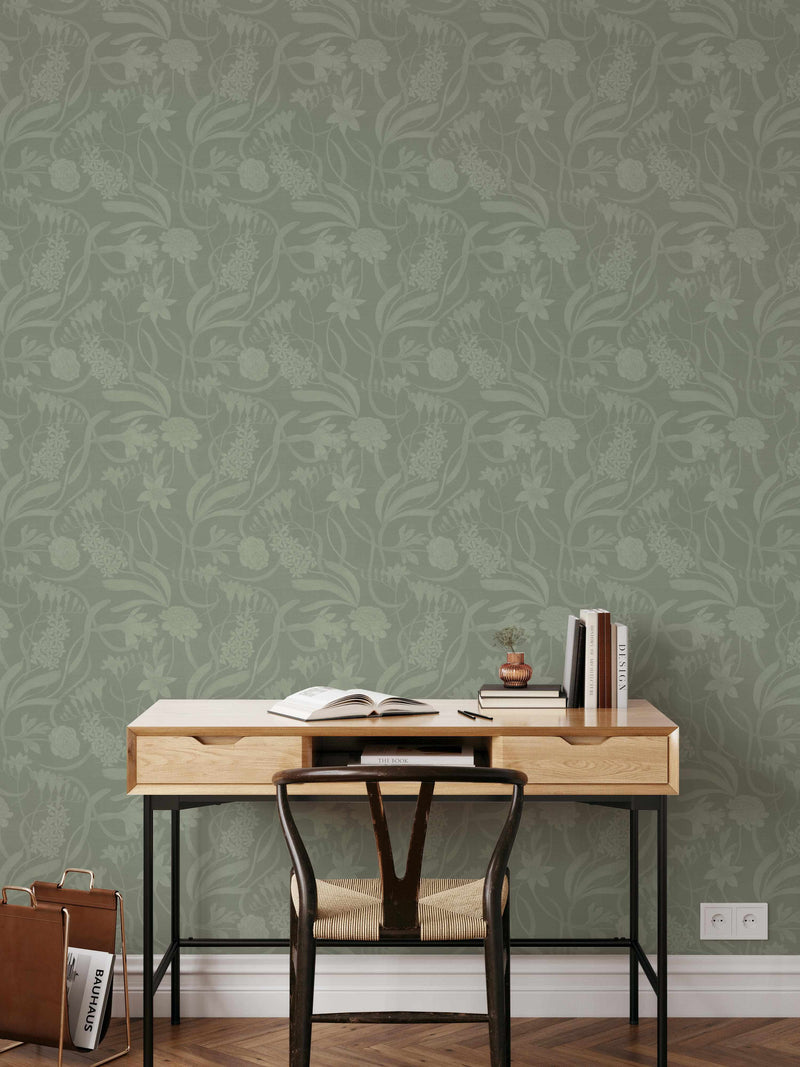In this image, a cozy, light wood desk with black metal legs is placed against a wall. The desk is compact, featuring two drawers and is adorned with several items. An open book rests on the desk, accompanied by a stack of books standing upright and a few pens. A small bonsai tree adds a touch of greenery beside the books. A smaller golden container is visible on the desk. Adjacent to the desk, a matching black metal chair with a woven wicker seat sits invitingly.

The background showcases a sophisticated wallpaper with sage green tones and a floral pattern. A dual-sided electrical outlet is situated just above the white crown molding on the lower right side of the wall. On the floor to the left of the desk, there is a brown vinyl record holder with gold handles, containing a record that reads "Bauhaus." The overall scene exudes an elegant European style, with a serene and organized workspace complemented by the rich, patterned wallpaper.